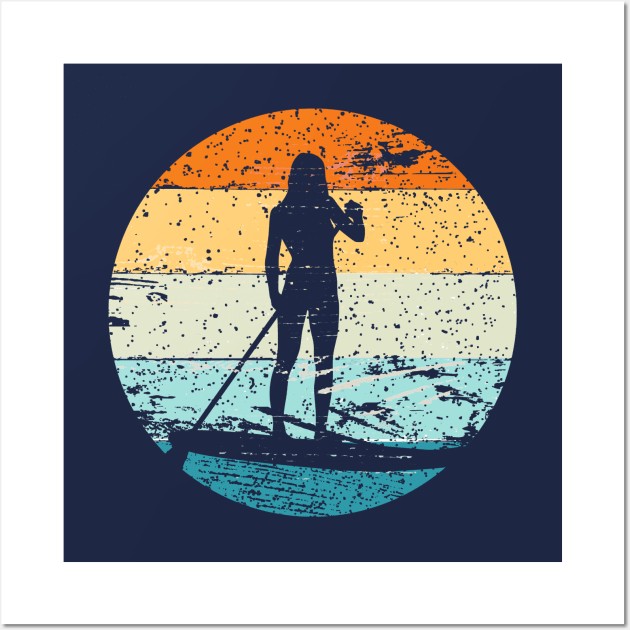This image features a distinctively stylized emblem, possibly resembling woodblock or vector art, set against a white background. In its core is a large dark blue square, containing a central circle divided into five horizontal bands of colors: vibrant orange at the top, followed by yellow, pale yellow, light blue, and darker blue at the bottom. Against these colorful stripes, reminiscent of a sunset with the lower blues symbolizing water, stands the dark blue silhouette of a woman on a paddleboard. She stands upright, gripping an oar that cuts through the vivid bands, suggesting motion through the calm waters. Adding to the rustic, aged aesthetic are scattered specks and scratches in dark blue, which overall provides a rugged, vintage look to the composition.